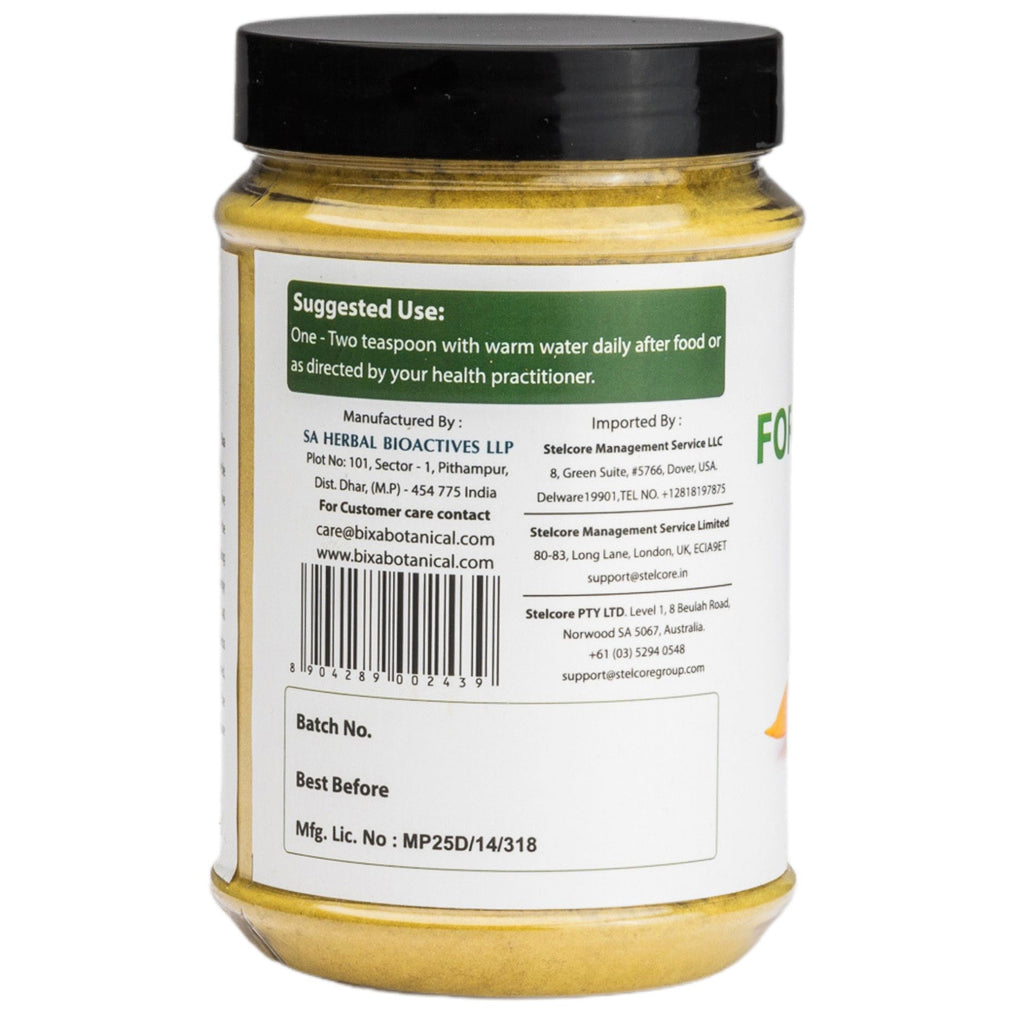This is an image showcasing the back of a transparent plastic jar containing a yellow powdered substance. The jar features a black cap and a detailed label with green and white accents. Prominently displayed in a green box at the top, the label specifies "Suggested Use: 1-2 teaspoons with warm water daily after food or as directed by your health practitioner." The adjacent sections provide additional information: on the left, it states the product is manufactured by S.A. Herbal Bioactives, LLP, Plot Number 101, Sector 1, Pithmapur, District Dhar, MP454775, India, along with customer care contact details at care@bixabotanicals.com and the website www.bixabotanicals.com. The right side details the importer, Stelcor Management Service LLC, with addresses in the U.S., London, and Australia. At the bottom, a rectangular box includes spaces for batch number, best before date, and manufacturer license number (MFG-LICNO-MP25D-14-318), though some fields are not filled out. The content of the jar, visible through the transparent plastic, reveals a striking yellow powder.